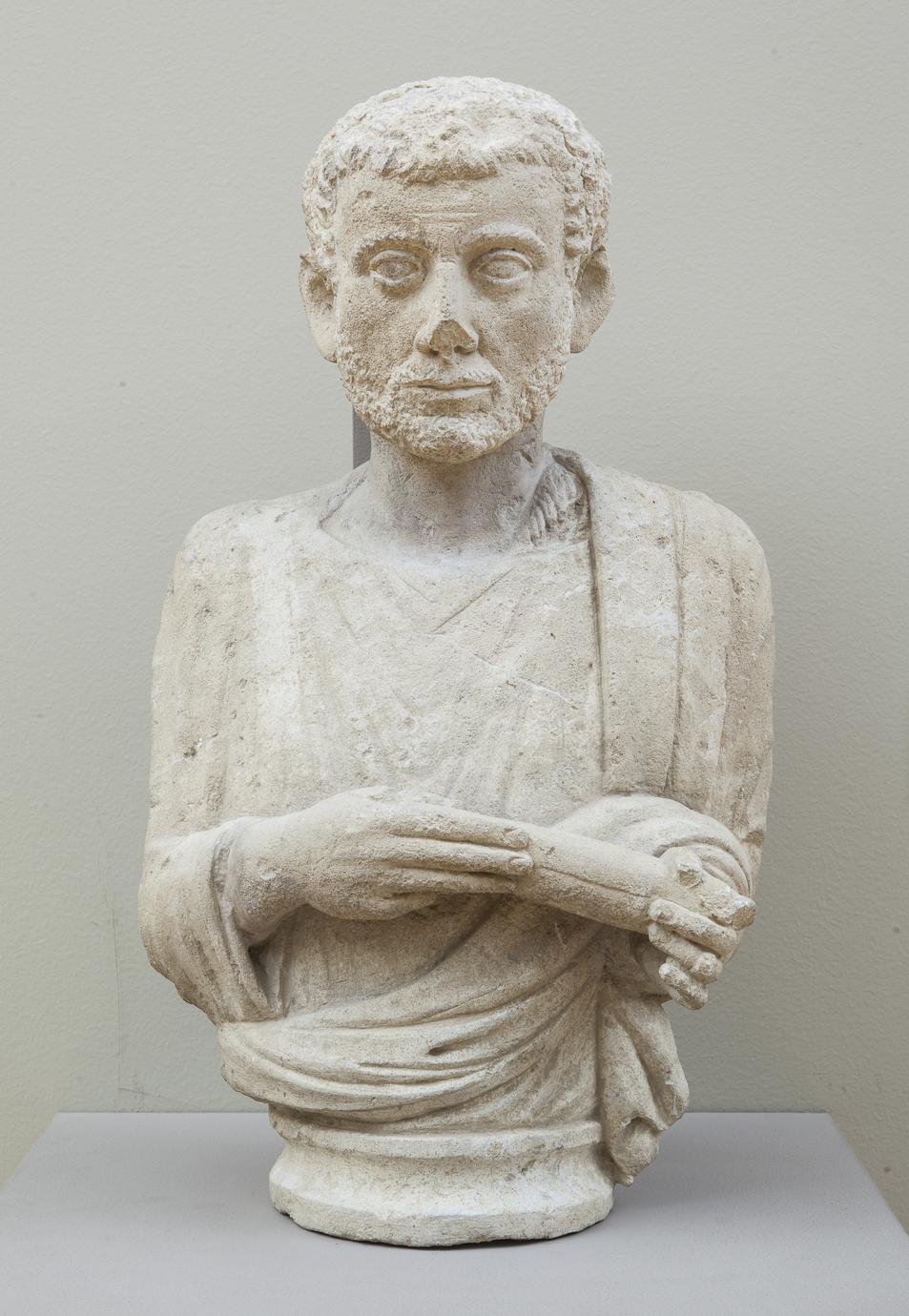This image features an off-white stone sculpture of a bearded man, set against a light green, almost olive backdrop. The figure, rendered from the torso up, appears to be from the Roman era. He has short, crew-cut hair and appears to be wearing a robe that drapes over his shoulder and arm. The sculpture is captivating in its details; his eyes, ears, and other facial features are clearly defined, with a notable chip on the nose's tip. His hands hold a cylindrical object, intricately carved to suggest significance. The statue rests on a round, flat base, placed on a white platform, which contrasts subtly with the backdrop. The piece is substantial, suggesting it could be displayed in a museum or as an impressive home centerpiece.